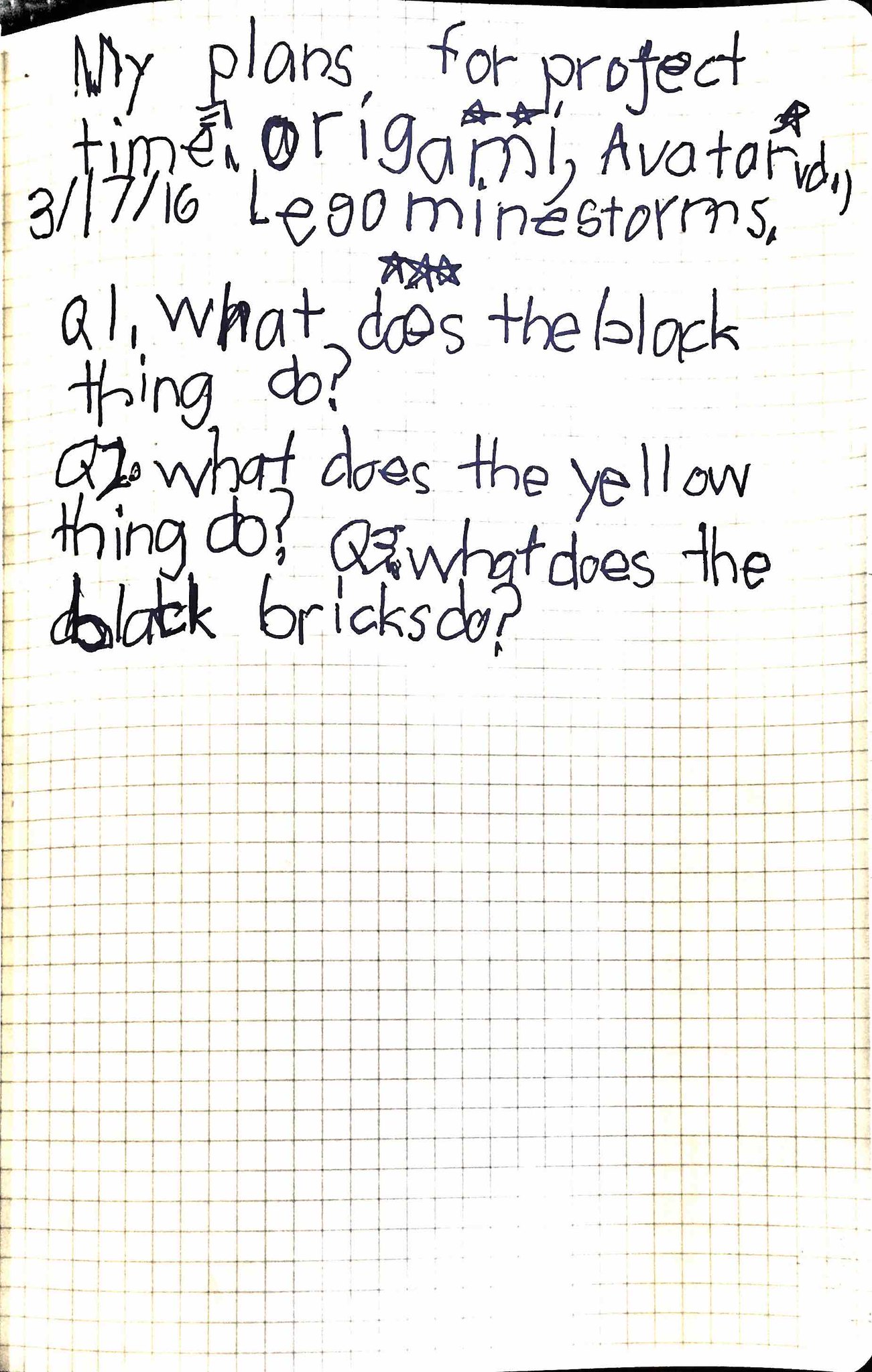This image showcases a slightly yellowed piece of graph paper filled with a child's handwritten note. The top portion of the paper is cluttered with disorganized and hard-to-read text, which appears to have been hastily penned. The note reads: "My plans for project time: Origami, Avatar, 3/17/16, Lego Mindstorms." Three stars are scattered around this section. Below this, three questions are listed: "Q1: What does the black thing do?" "Q2: What does the yellow thing do?" and "Q3: What do the black bricks do?" The overall presentation suggests this note was quickly put together, possibly for a school project or a child's personal reference, and subsequently set aside.